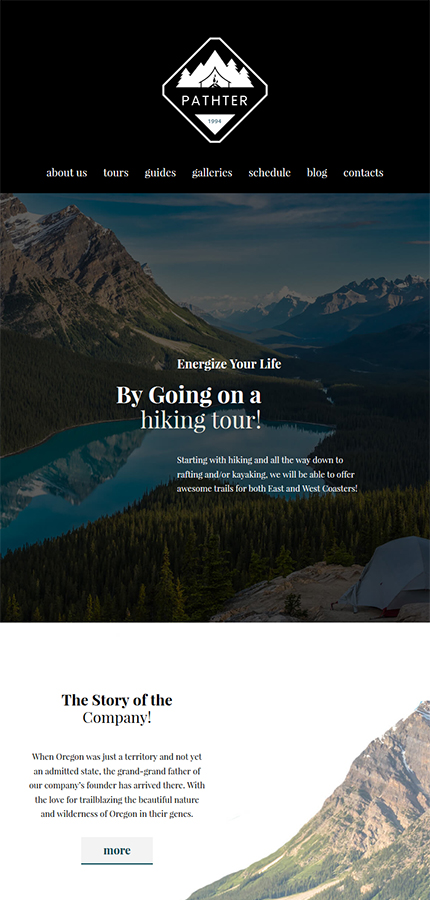At the top of the image, there is a logo featuring a forest and a house, accompanied by the text "Panther 1994." Below the logo, a navigation bar with tabs labeled About Us, Tours, Guides, Galleries, Schedule, Blog, and Contact is set against a black background.

The main picture depicts a breathtaking landscape where a serene river meanders through a dense forest. Forested areas stretch across both sides of the river, with majestic mountains rising in the distance, particularly prominent behind the forest to the left. The scene exudes an expansive and untouched wilderness.

Overlaying the landscape, there is text that reads: "Energize your life by going on a hiking tour. Start with hiking and progress all the way to rafting or kayaking. We offer remarkable trails for both east and west coasters."

Below this section, a white background frames another part of the webpage. In the right-hand corner, there is an image fragment showing a mountain and a trail. Adjacent to the image, more text narrates the company’s history: "When Oregon was just a territory and not yet an admitted state, the great-grandfather of our company's founder had arrived there with a love for trailblazing the beautiful nature and wilderness of Oregon coursing through their genes." A "More" link, underlined, invites users to delve deeper into their story.